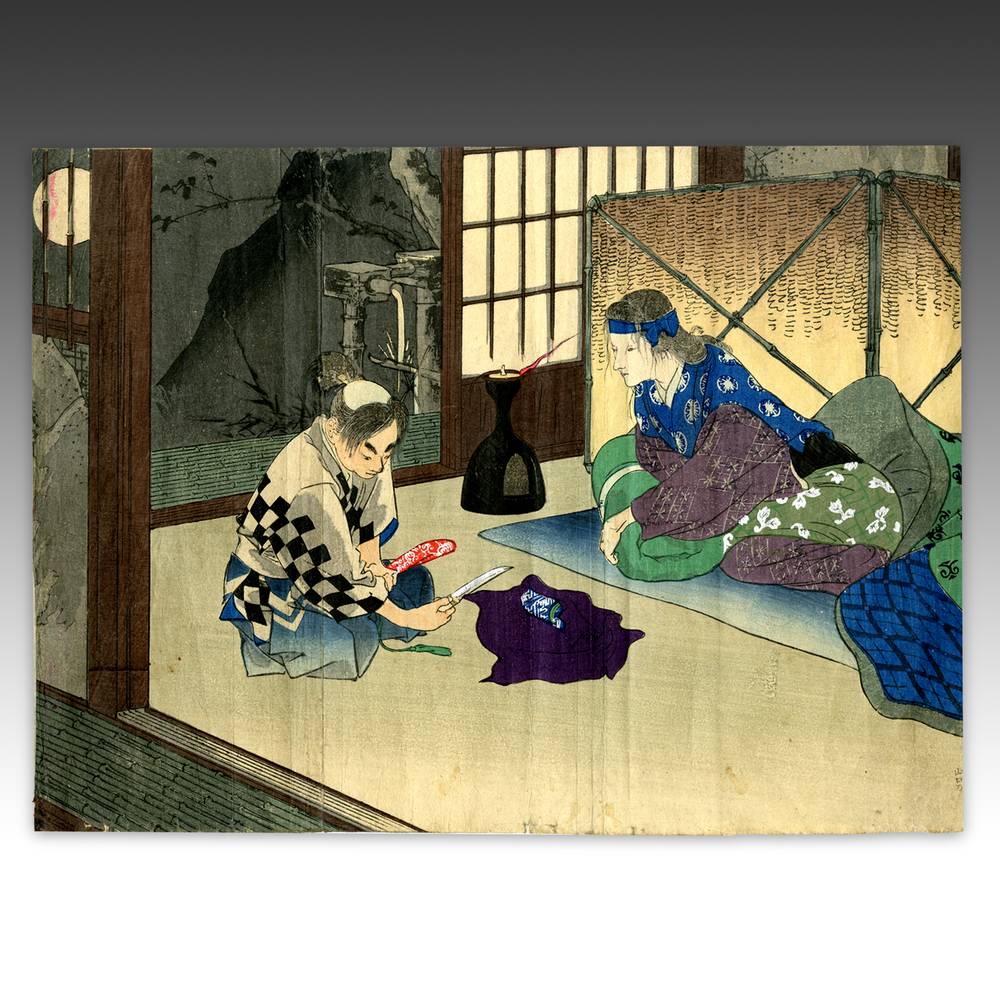The image is a traditional Japanese painting, displayed on a dark grey wall that fades to white at the bottom. The painting depicts two individuals seated on a beige and green tatami mat inside an open hut with visible dividers. The individual on the left, who appears to be Asian, is seated cross-legged and holding a short white dagger with a red decorative sheath in one hand and a red and white fan in the other. This person is clad in a white kimono with black checkered sleeves, blue interior sleeves, and cyan leggings. Their hair is styled in a traditional samurai fashion, and they are looking intently at the dagger. The space in front of them features a purple cloth with a patterned cloth inside it.

The individual on the right appears to be a woman with lighter skin and black hair held back by a blue bandana. She is dressed in a blue kimono adorned with circular symbols and accented by purple sleeves and a bottom section. She is leaning against a green blanket that is decorated with white flowers and is partially covered by another intricately embroidered blue and green blanket. She is observing the person on the left with a contemplative expression, her position slightly supported by the green blanket. Additionally, there is a black incense pot, shaped like an upside down chalice, placed beside the blankets.